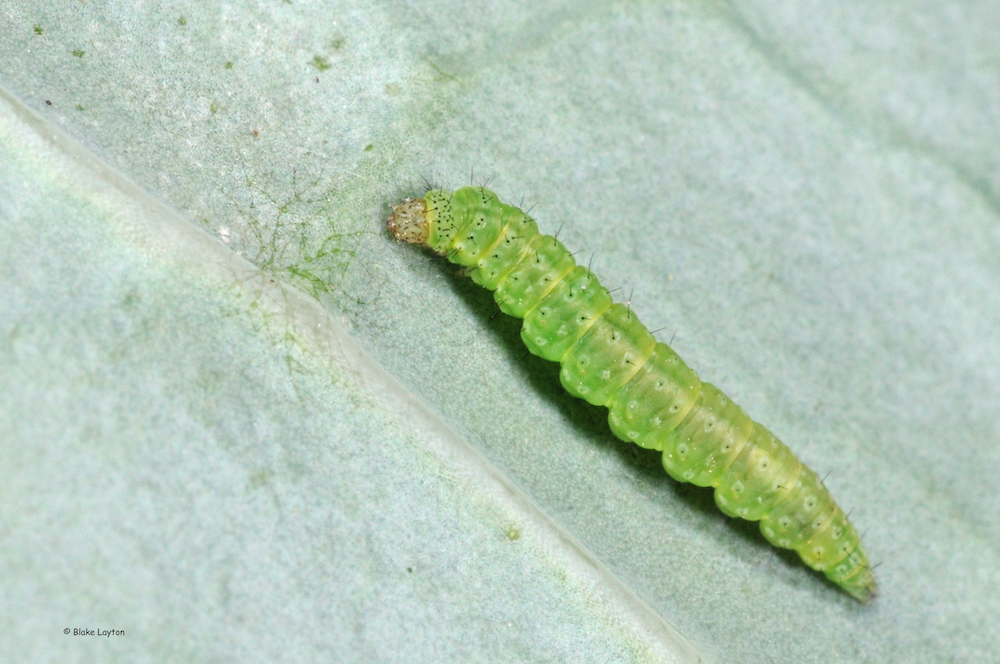A close-up photograph of a vibrant light green caterpillar crawling across a light bluish-green leaf with distinct indentations. The caterpillar, with its beige head and small brown nose or mouth, is detailed with numerous small hairs along its body and head. Each segmented part of the caterpillar's body features lighter green spots with central black hairs, forming a paired pattern down its back. The leaf exhibits a small green splotch near the caterpillar and beige creases. The caterpillar's body also reflects a golden hue where the light strikes it directly. In the bottom left-hand corner, the image is marked with the copyright notice "Blake Leighton," acknowledging its photographer. The scene is brightly lit, emphasizing the caterpillar's unique details and the subtle shadows it casts on the leaf.